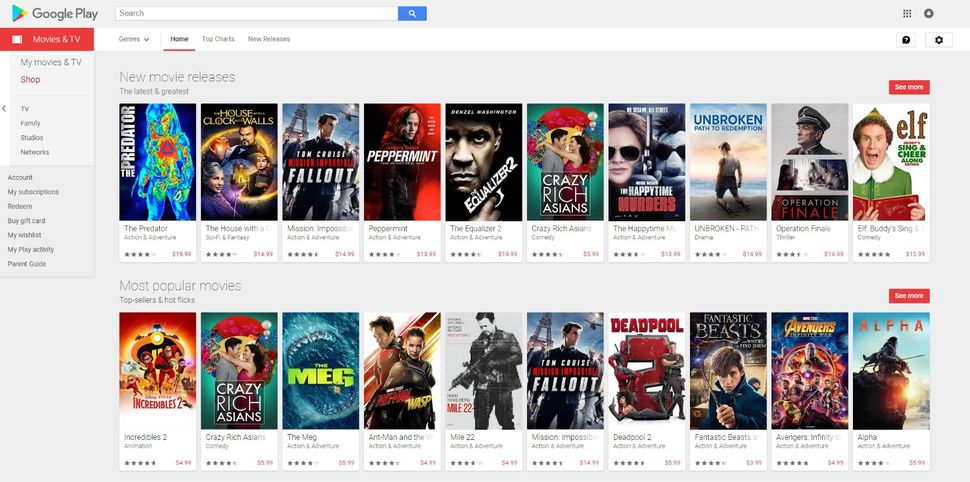In this image of the Google Play Store, the background is a light gray color. In the upper left corner, the Google Play logo is prominently displayed alongside the text "Google Play." To the right of the logo, there is a search bar available for users to look up specific content. Along the left side of the screen, various tabs and categories can be seen, indicating different sections of the store.

On the right side, the store showcases a selection of movies in two distinct rows. Starting from the top row, the movies displayed include "The Predator," "Mission: Impossible - Fallout," "Peppermint," "The Equalizer 2," "Crazy Rich Asians," "Unbroken: Path to Redemption," and "Elf." The bottom row features "Incredibles 2," "Crazy Rich Asians" again, "The Meg," "Mission: Impossible - Fallout" again, "Deadpool 2," "The Avengers," and "Alpha." Each movie listing includes its title, a price, and a star rating.